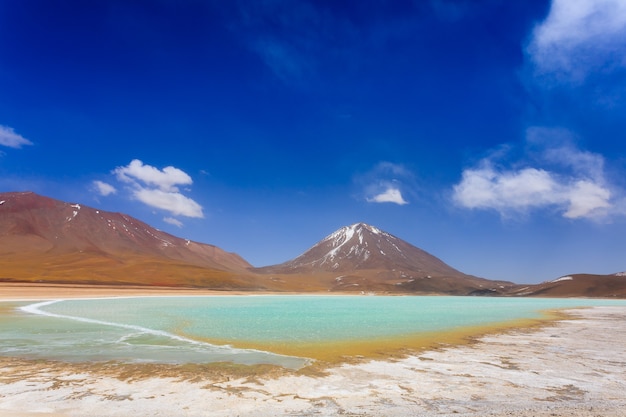This captivating image portrays a serene and picturesque landscape that melds a variety of natural elements. Dominating the top of the picture is a vibrant, clear blue sky dotted with a few patches and clusters of white clouds. Below the sky, spanning the middle of the image, lies a striking body of teal-green water, bordered by a mix of golden yellow and white sand. The water's surface showcases gentle ripples and foamy waves, creating a calming effect. Further back, majestic mountains and hills rise, their peaks varying in shape with one notable sharp peak on the right and another broader, flatter mountain. Snow caps are visible on these distant mountains, adding contrast to the warm colors of the sand and earth below. Altogether, the scenery combines deep blues, earthy browns, bright golden sand, and the sea's characteristic green, crafting an idyllic and tranquil outdoor scene.